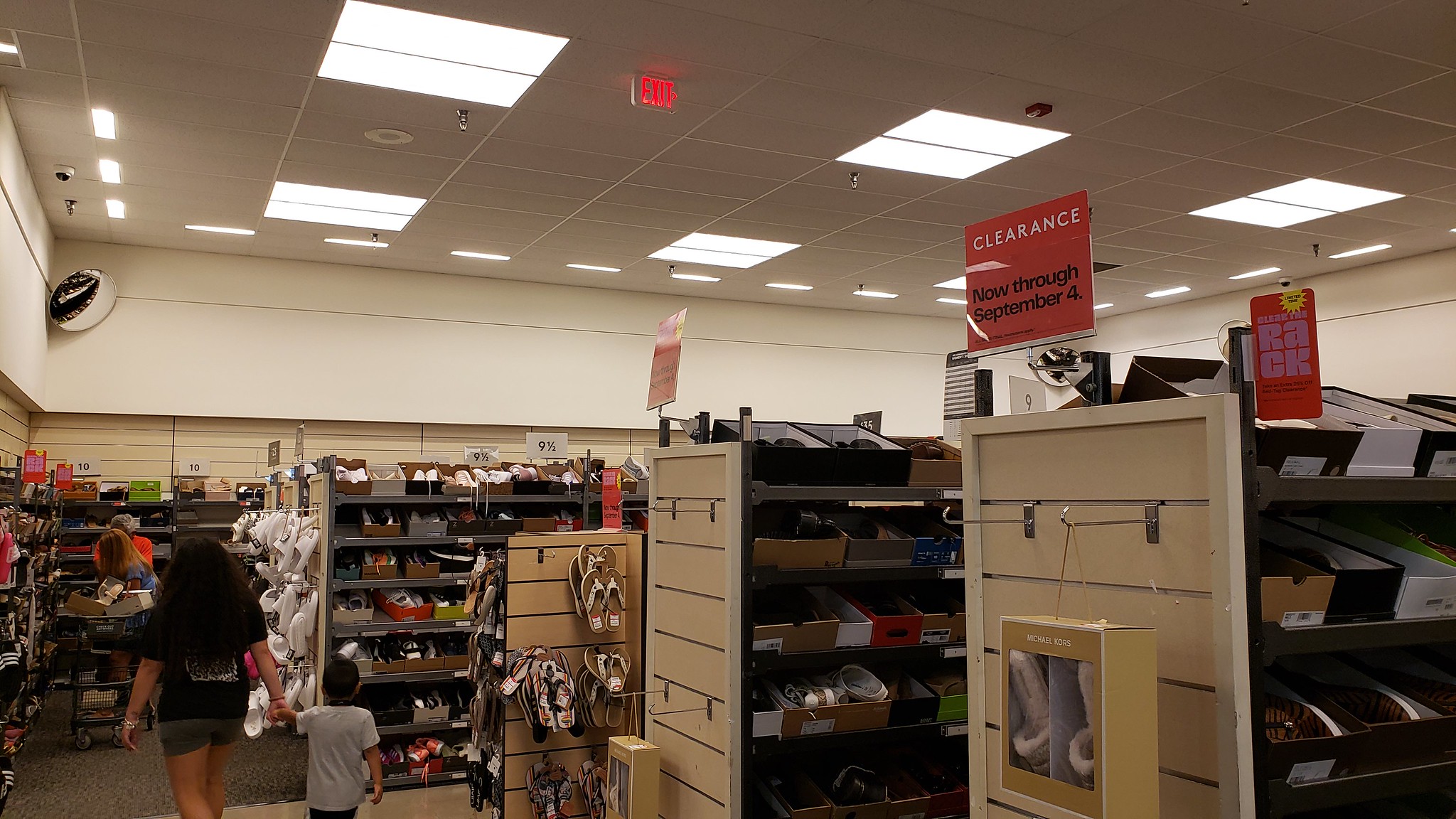The colour photograph depicts a bustling shoe store mid-clearance sale, with a red sign prominently displaying "CLEARANCE" in white letters and “now through September 4th” in bold black text. The scene is taken inside an aisle, with numerous shoe boxes helter-skelter on metal racks, some opened and others askew, enhancing the overall disarray. Visible on the right end cap, a variety of shoes, flip-flops, and slippers dangle from metal hangers, while the left end cap has a nearly empty display with a collection of white slip-on sandals. In the background, one can observe customers, including a girl with long hair wearing shorts, holding the hand of a young boy as they navigate the cluttered store. The store’s infrastructure is visible with ceiling tiles, lights, a camera, a sprinkler system, and an exit sign, adding to the mundane reality of a busy retail environment.